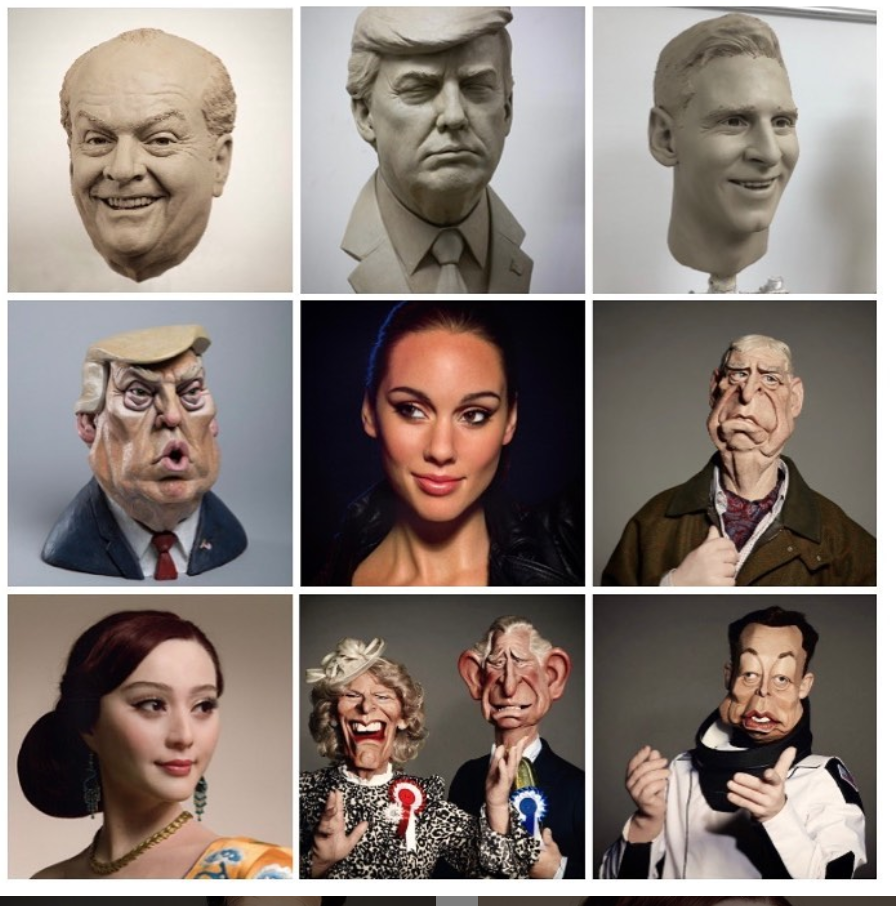This image is a three-by-three grid featuring nine photographs of sculptures and caricature busts of various famous individuals, predominantly depicted in either a realistic or exaggerated style. In the top row, from left to right, are three gray clay sculptures: the first is a smiling, bald white man, possibly Jack Nicholson; the middle one resembles Donald Trump with his eyes closed; and the third is a smiling man with hair, potentially Lionel Messi or another famous figure. The second row is composed of colored sculptures: on the left is a vibrant caricature of Donald Trump in a speaking pose; the middle features a photograph of a woman with black hair, possibly an actress like Natalie Portman; and the right depicts a detailed sculpture of an elderly white man in a brown jacket and a white collared shirt holding his lapel. The bottom row includes: on the left, what appears to be a color photograph of a Chinese actress such as Fan Bingbing; the middle shows caricature sculptures of King Charles and Camilla; and the rightmost is a character sculpture of a priest in white robes with a large black collar, possibly resembling Elon Musk. Each piece varies in realism and caricature style.